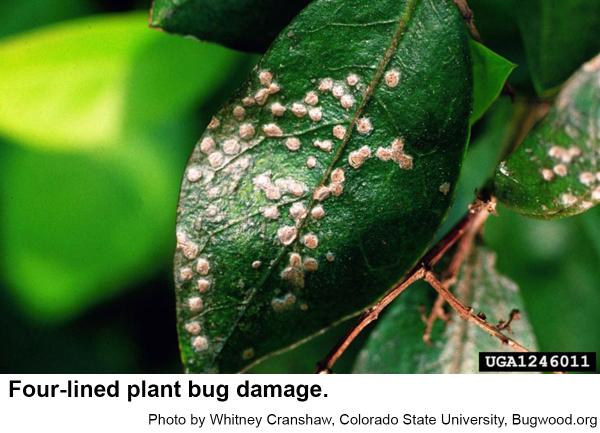This close-up daytime photograph showcases a pair of dark emerald green leaves bearing significant damage caused by four-lined plant bugs. Tiny, rust-colored spots are scattered across the leaves, evidence of the bug damage. The leaves, attached to dark brown stalks, are bathed in sunlight, with a backdrop of blurred, light green foliage that highlights the clarity of the damaged leaves in the foreground. Notably, another leaf at the top also displays similar damage. The photograph, captured by Whitney Cranshaw from Colorado State University and shared on bugwood.org, is labeled with the identifier UGA 1246011.